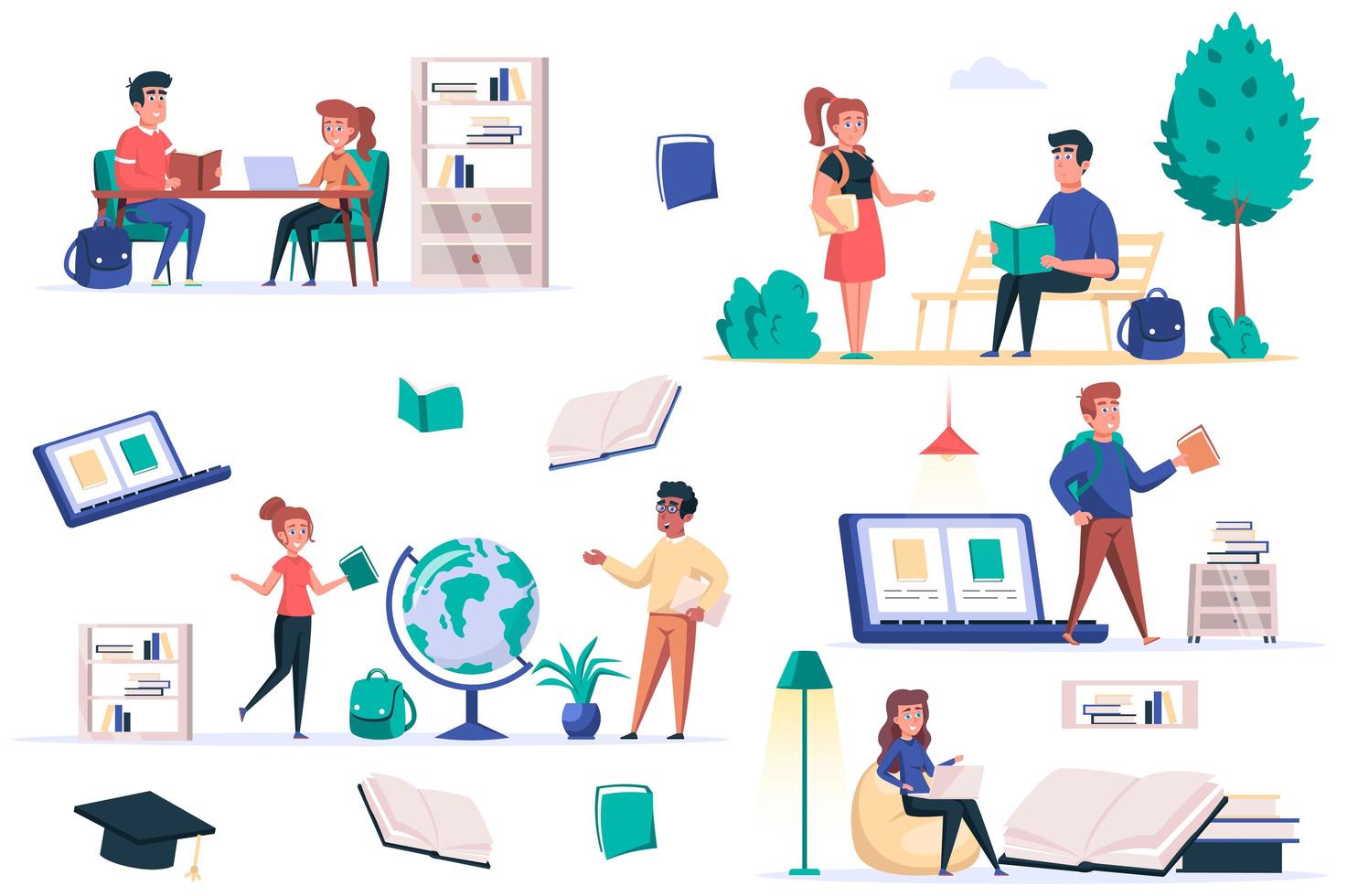The illustration is a collage of scenes that depict various academic and leisure activities common in a student’s life, all arranged within a horizontally-oriented rectangular frame.

In the upper left corner, two students, a boy and a girl, are engaged in study at a table that holds several books, suggesting an environment that could be either an office or a library. The boy has a backpack, hinting at a high school or college setting.

In the upper right corner, the same pair appears to have moved outdoors to a park. The girl carries a book while the boy reads on a park bench near a small tree, highlighting a blend of academic and relaxed activities.

Mid-row on the left, the scene shifts to a large globe where the boy and girl stand. The girl, with a turquoise backpack, listens as the boy talks, likely discussing geographical topics. A small bookshelf nearby adds to the academic ambiance.

A standalone row in the upper area features items indicative of study: a laptop, a book, and an open notebook. Adjacent to this, a man speaks in what appears to be a library setup. He is near a roller shelf with drawers filled with books, and a ceiling-mounted lamp illuminates the area.

On the bottom row, various educational symbols are depicted: a graduation cap, an open book, and a closed bluish-green book, symbolizing the journey of learning and achievement.

In the lower right corner, a girl with a blue shirt sits comfortably on a brown beanbag chair. She uses a laptop, surrounded by an open book and a stack of books, under the light of an aqua-colored desk lamp, showcasing a cozy study nook.

Each vignette in this collage collectively presents a rich narrative of student life, merging studies with everyday activities.